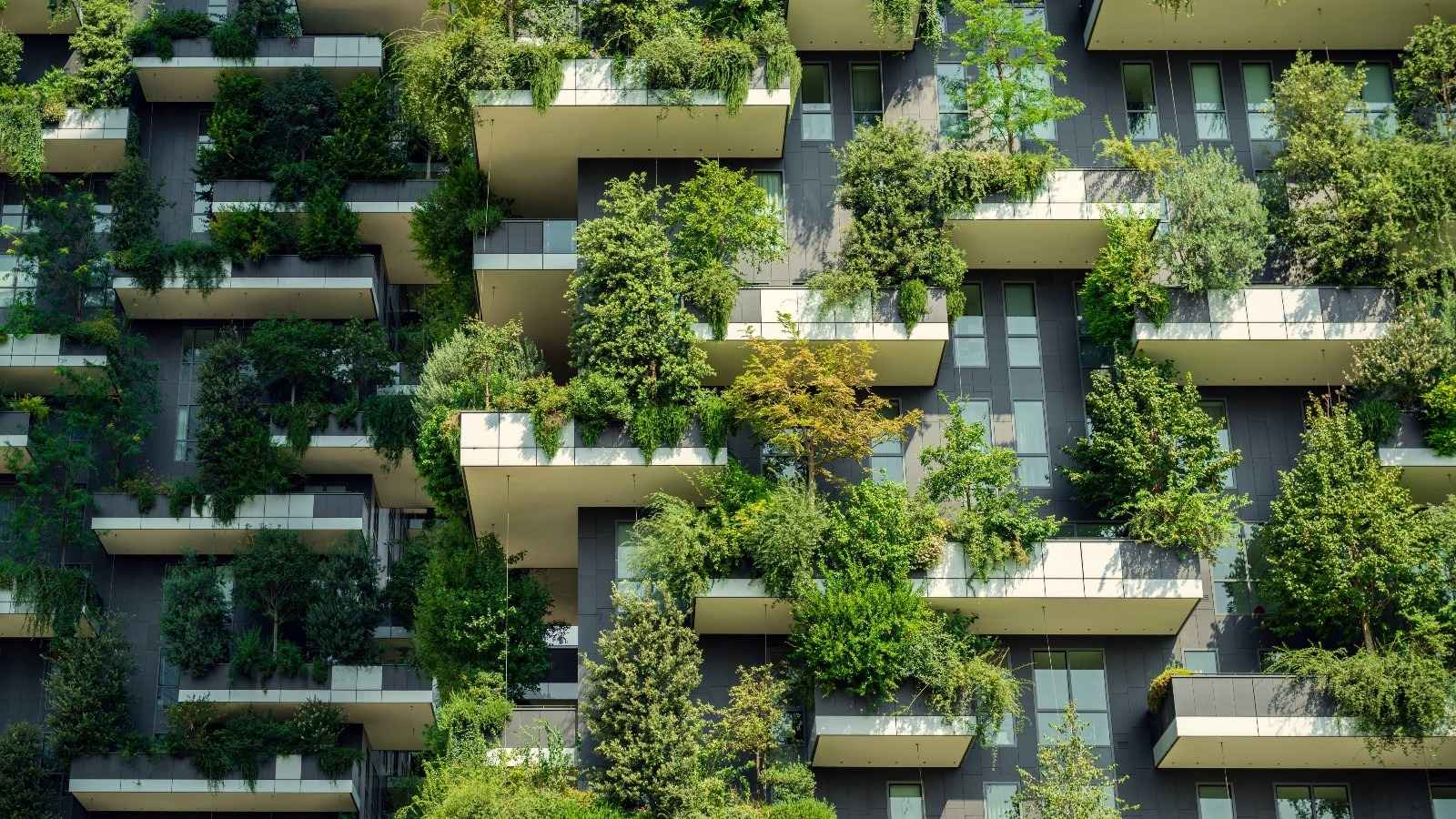The image showcases an exterior shot of a tall, sleek, and futuristic building, positioned in a cityscape. The building facade is characterized by a sophisticated blend of gray and white tones. Most prominently, it features an intricate array of balconies that jut out irregularly, each overflowing with lush, vibrant green foliage, likely small trees. This abundance of greenery spills over the edges of each balcony, contributing to a strikingly verdant appearance. The balconies and greenery are a dominant visual element, capturing the viewer's attention. The building sports numerous vertically oriented windows, many of which are double or quadruple paned. The perspective of the image suggests it was captured from a high vantage point, offering a comprehensive view of these balconies and their overflowing greenery, set against the dark gray and white backdrop of the building. The entirety of the visible image is composed of the building facade, punctuated by the bright green canopies of the trees, the white balcony undersides, and the consistent, orderly placement of windows.